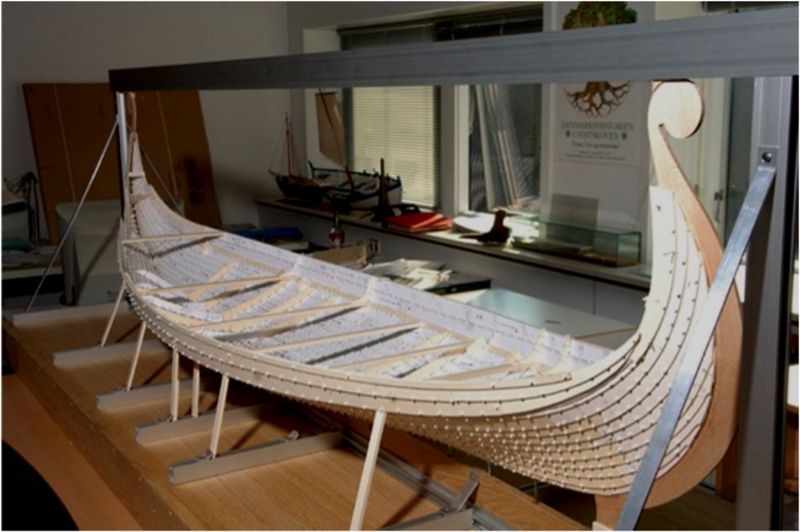The image captures an indoor scene, possibly within a museum or an office space dedicated to boat restoration or display. The setting features white walls adorned with various signage and shelving, along with blinds drawn over the windows. Multiple boxes containing assorted items are visible, contributing to the workspace ambiance. 

The focal point of the image is a meticulously mounted old canoe-like boat. Suspended within a rectangular gray metal frame, the boat exhibits elegant craftsmanship. Its structure is primarily light brown wood with horizontally placed boards inside that seem designed for seating. The boat's ends curve upward and form rounded points, adding to its ornate appearance. The exterior bottom of the boat is a darker brown, providing a rich contrast to its lighter interior. Beside the display, a wooden board is seen hanging on the side wall, complementing the boat's classic aesthetic. The steel beam structure holding the boat suggests an environment where historical preservation or detailed crafting of boats is a primary focus.